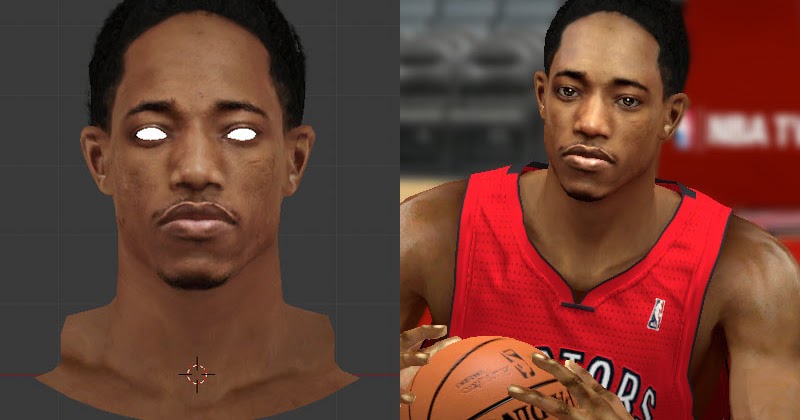The image consists of two separate computer-generated shots of a character who appears to be a player in a video game. 

On the left, there's a detailed headshot of a black man with short black hair and a large forehead. His eyes are whited out, and the image focuses on his collarbone, neck, and face. You can clearly see his well-defined facial features, including his eyebrows, nose, a little mustache, lips, goatee, and ears. A centering icon and a faint graphic background further characterize this depiction.

On the right side, the same character is shown from the torso up, this time in a red uniform top while holding a basketball. The background showcases empty seating and a red banner, devoid of any people. This image reveals his eyes, which were obscured in the previous shot, and presents him with a sad expression, giving a plain or distant stare.